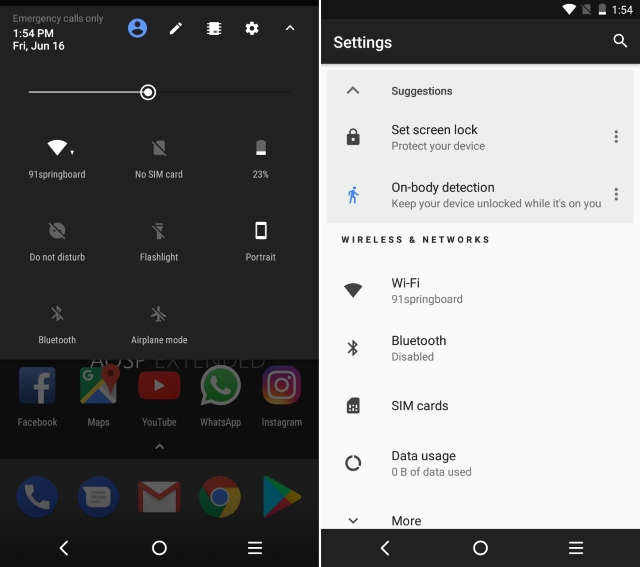**Detailed Caption:**

This is a comprehensive screenshot from a mobile device running on the Android operating system. The image displays two screens side by side.

The left screen shows the device's notification shade or quick settings panel. At the top, the status bar indicates "Emergency calls only," with the current time displayed as 1:54 PM and the date as Friday, June 16th. The screen brightness slider is positioned slightly below the midpoint, indicating moderate brightness. Noticeable icons include the profile button, a pencil icon for editing, a gear icon for settings, and another icon resembling film from a film camera. The connected Wi-Fi network is labeled "91 springboard," the device shows a status of "No SIM card," and the battery percentage is at 23%. Additional settings indicate that "Do Not Disturb" mode is off, the flashlight is off, the device is in portrait orientation, Bluetooth is turned off, and airplane mode is also off. In the background, various app icons are visible, including Facebook, Google Maps, YouTube, WhatsApp, Instagram, along with core applications like Phone, Messaging, Email, Google Chrome, and the Google Play Store.

The right screen displays the device's settings menu with the "Suggestions" section at the top, highlighting options like "Set screen lock" and "Protect your device." The "On-body detection" feature is also suggested, identifiable by a small blue icon of a person. The available settings options include Wi-Fi (enabled), Bluetooth (disabled), SIM cards, and data usage, which shows zero data used so far. Each setting's status is clearly indicated, providing a thorough overview of the device’s configurations.

This detailed combination of screens provides an insightful glimpse into the device's operational status and user settings.